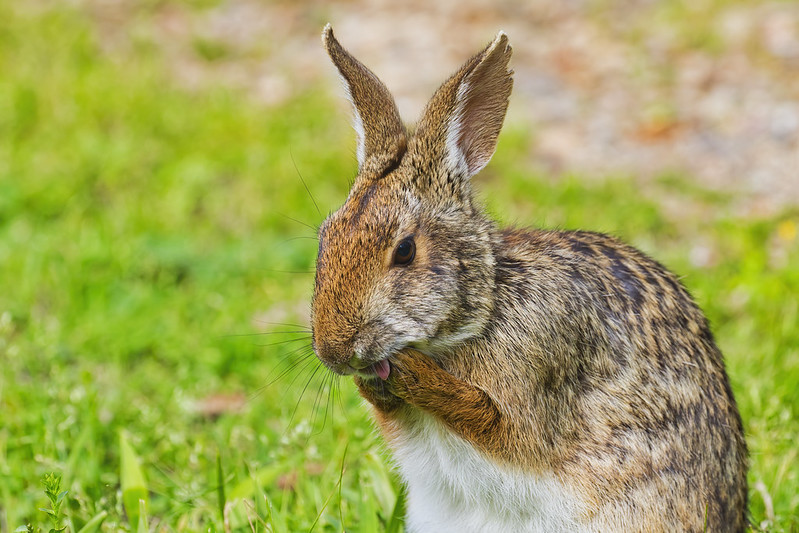This close-up photograph features an adorable multicolored rabbit positioned in the bottom right-hand corner of the frame, adhering to the rule of thirds in photography. The background is artfully blurred, showcasing a strong bokeh effect that highlights the rabbit as the main focus. The ground beneath the rabbit is filled with lush green grass, while further back, the colors shift to brown, possibly indicating dead grass, leaves, or a dirt patch.

The rabbit itself boasts a unique fur pattern: its belly and the edges of its ears are white, while the top of its coat displays a mix of light brown with black stripes and spots. This color combination creates an interesting texture across its body. Notably, the rabbit's small pink tongue is visible as it sticks out slightly, adding a cute and engaging element to the image. Its brown eyes are gazing intently, contributing to the overall warm and natural feel of the photograph.

The rabbit's front paws are adorably pressed up against its mouth, seemingly holding a pink flower petal, which it appears to be eating. This detail adds an extra layer of charm and liveliness to the scene. The setting appears to be outdoors, possibly in someone's yard, where the background elements, although blurred, hint at a natural environment with varying shades of green and brown.